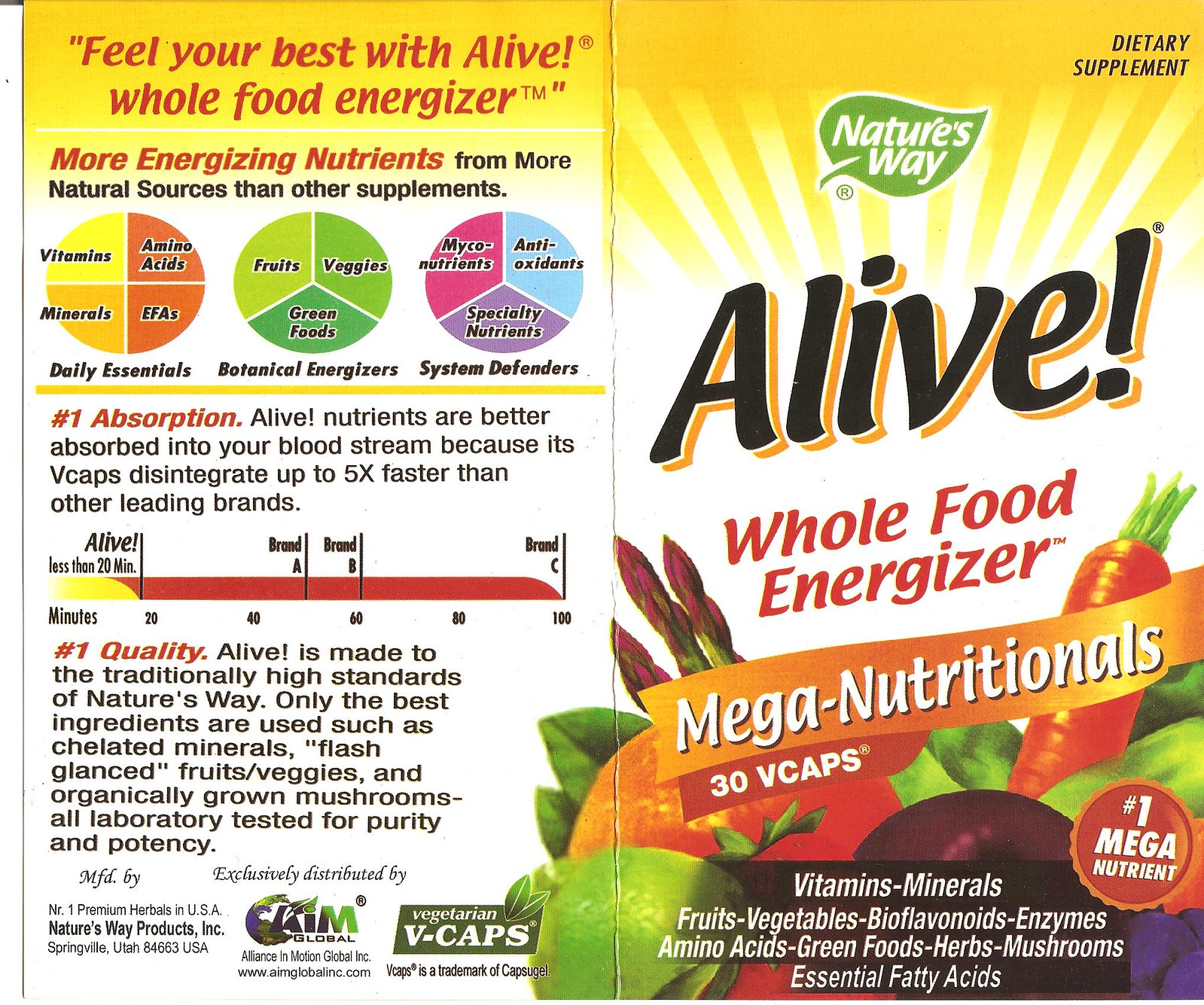The image depicts a flattened, torn-open box that originally contained dietary supplements. On the right-hand side, the packaging prominently displays the text "Dietary Supplement" and "Nature's Way," written within a green leaf in white letters. The product name "ALIVE" is presented in bold black letters with an orange shadow and an exclamation point. Below that, it describes the product as a "Whole Food Energizer" with "Mega Nutritionals," containing "30 V-caps."

The box highlights that this is the "#1 Mega Nutrient" and lists its ingredients, including Vitamins, Minerals, Fruits, Vegetables, Bioflavonoids, Enzymes, Amino Acids, Green Foods, Herbs, Mushrooms, and Essential Fatty Acids. It also boasts that "Alive Nutrients are better absorbed into your bloodstream because V-caps disintegrate up to 5 times faster than other leading brands." The packaging emphasizes that it is "#1 in Quality."